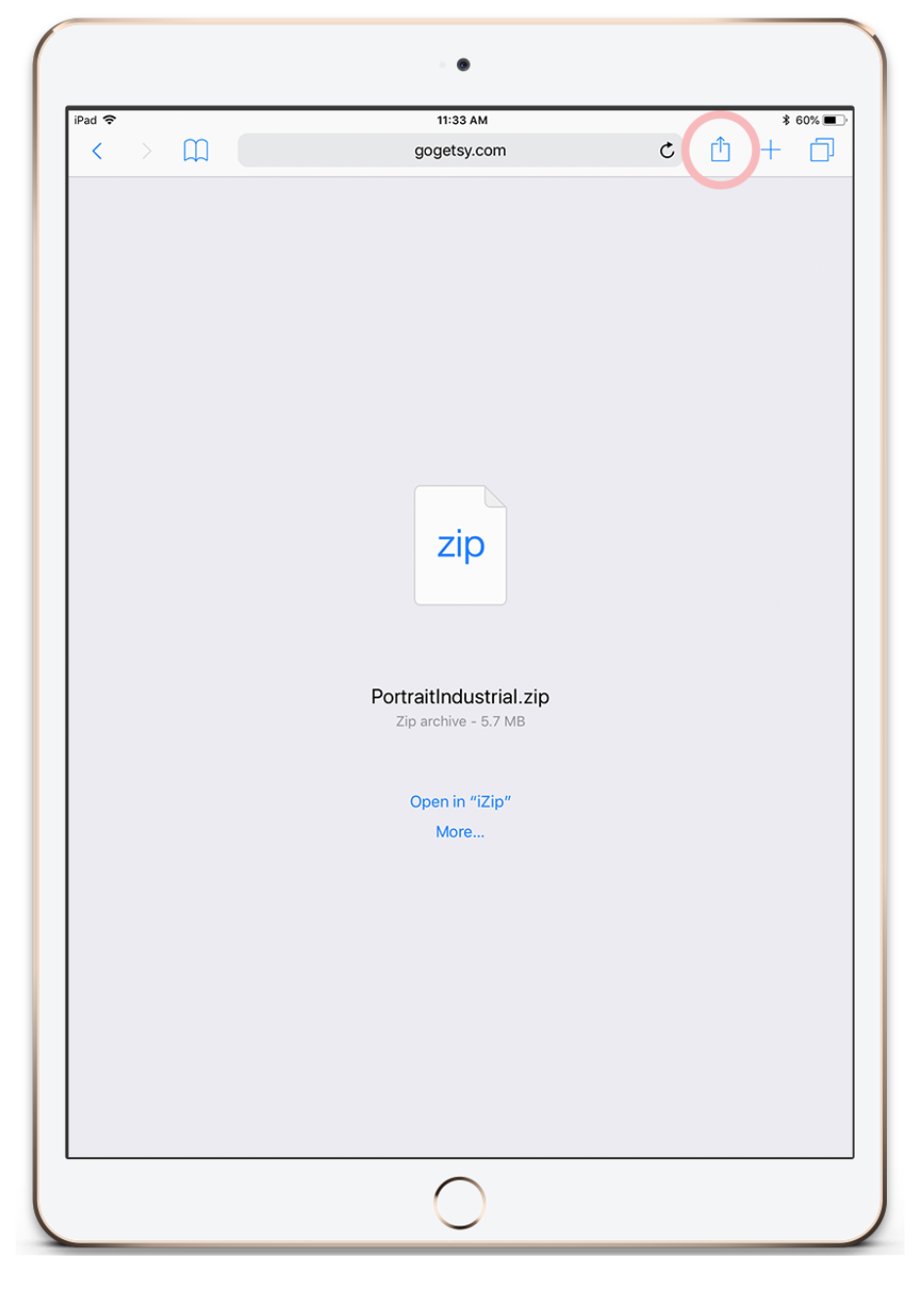The image displays an iPad screen with various elements visible, implying the device is being used in real-time. At the top-left corner, the word "iPad" is displayed alongside a wireless signal icon. Centrally located on the screen, the time reads "11:33 AM." Fairly top-right, the battery percentage is indicated as "60%" with the accompanying battery icon and a Bluetooth symbol.

Immediately below this header information, there is a blue arrow pointing left and a gray arrow pointing right. Highlighted in blue is an "Open Book" icon. An address bar follows, containing a web address, features a pink circled box with an upward-pointing arrow protruding from it, symbolizing a sharing option. Adjacent to this is a blue plus sign and two overlapping boxes, perhaps indicating tab management.

The majority of the page consists of a gray background. Centrally located within this gray expanse is an image of a document with a folded corner, displaying "Zip" in blue text. Below this, the text "Portrait Industrial.zip" is printed in black, with "Zip Archive 5.7 megabytes" in gray below it. Further down, the options "Open in iZip" and "More…" are presented in blue text.

At the very bottom of the screen, the characteristic circular home button, common to many iPad and iPhone models, is visible.